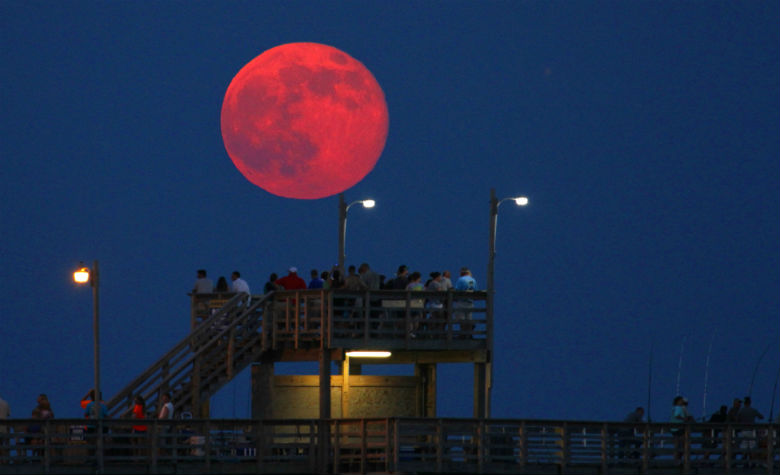The image captures a bustling nighttime scene on a wooden pier under a striking blood moon. The sky is a deep, dark blue, illuminated by the large, intensely red moon that dominates the horizon. A wooden railing runs along the pier, which features two distinct levels: a main boardwalk area and an upper deck reached by a stairway on the left. This upper deck or small second floor is crowded with around twenty people, all seemingly captivated by the extraordinary lunar spectacle. Some people on the lower boardwalk and the upper deck are leaning against the wooden fence, with a few on the bottom right engaged in fishing. Various light sources, including yellow lights on poles, street lamps, and a fluorescent light, create a soft glow across the scene. The overall atmosphere is serene yet lively, as people gather to witness the magnificent blood moon shining brightly overhead.